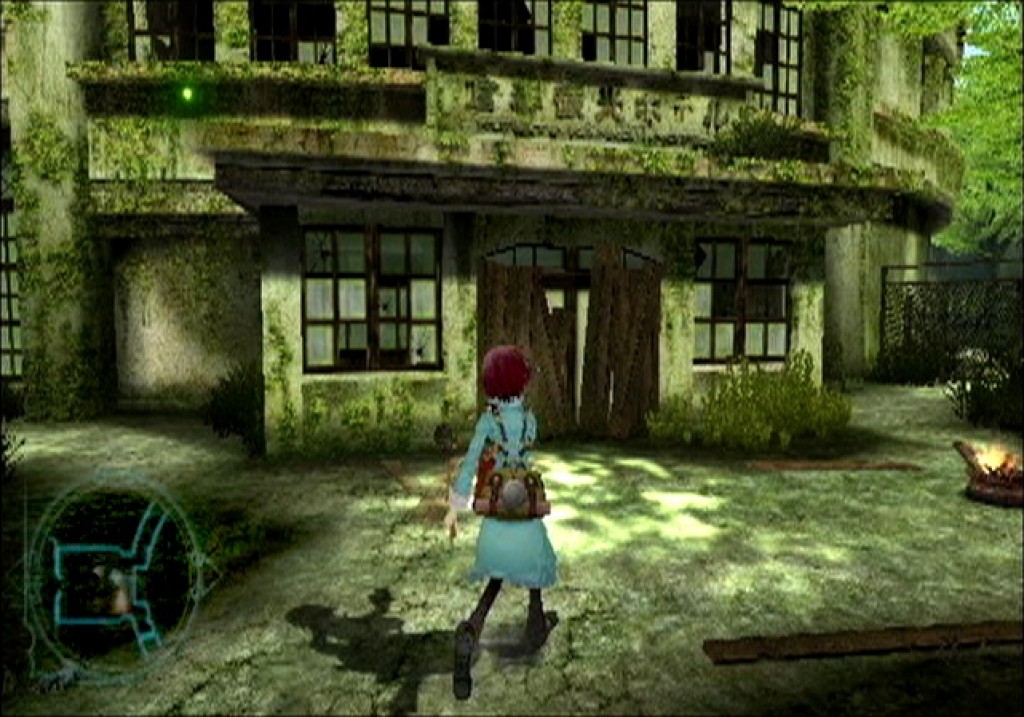This atmospheric photograph captures a scene of an ancient, moss-covered building nestled among trees. The structure appears to be several stories tall, with an overhang sheltering the front door and two flanking windows. Higher up, there are what seem to be balconies on the upper floors. The dappled sunlight filters through the canopy, casting a gentle glow into the yard. A lone figure, a woman with dark hair, strides confidently across the yard. She is wearing a blue coat and dark pants, carrying a large satchel on her back. The façade of the building is adorned with Chinese or Oriental characters, hinting at its heritage. The pervasive moss and overall state of neglect give the building a hauntingly beautiful look.